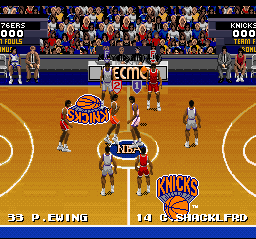The image is a frozen screen from an early basketball video game, likely from the mid-1980s, featuring the New York Knicks. The court is depicted with detailed lines and circles, and the Knicks logo is prominently displayed at center court where the tip-off is set to occur. The players Patrick Ewing (#33 in white) and Chris Shackelford (#14) are lining up for the jump ball, with the game score at 0-0. The game has not started yet. The background shows an audience and two large scoreboards, adding a realistic touch to the scene. Familiar elements suggest this could be a Tecmo game, evidenced by the Tekmo signage subtly visible in the background. The game captures the vintage essence of 1980s basketball video games with its graphics and team setup.